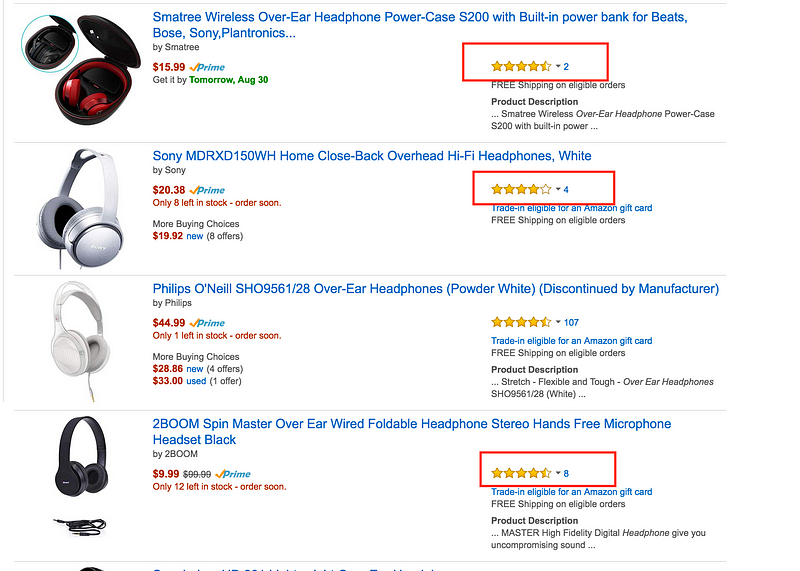The image displays a selection of headphone and earbud products, prominently featuring four different items. At the top-left, the headline reads, "Smarty Wireless Over-Ear Headphone Power Case S200 with Built-in Bank for Beats." The red case is open, revealing the red headphones inside, priced at $15.99. It also indicates that the item is eligible for Prime shipping with a delivery date of August 30th. 

To the right is a product box highlighted in red, showing a 4.5-star rating. Below it, a dropdown menu offers options such as "Free Shipping" or "Eligible Orders." The product description reiterates the name: "Smarty Wireless Over-Ear Headphone Power Case S200 with Built-in Power."

Next, the image features another set of headphones, the "Sony MDR-XD," priced at $20.38 with Prime. This product also has a rating of four stars and more buying options available, including eight offers from new sellers.

Further down, the "Philips O'Neill Headphones by Philips" are priced at $44.99 with Prime and hold a 4.5-star rating. 

At the bottom of the image, partially cut off, is the "Tube Boom Spin Master Over-Ear Wire Foldable Headphones," priced at $9.99 with a 4.5-star rating.